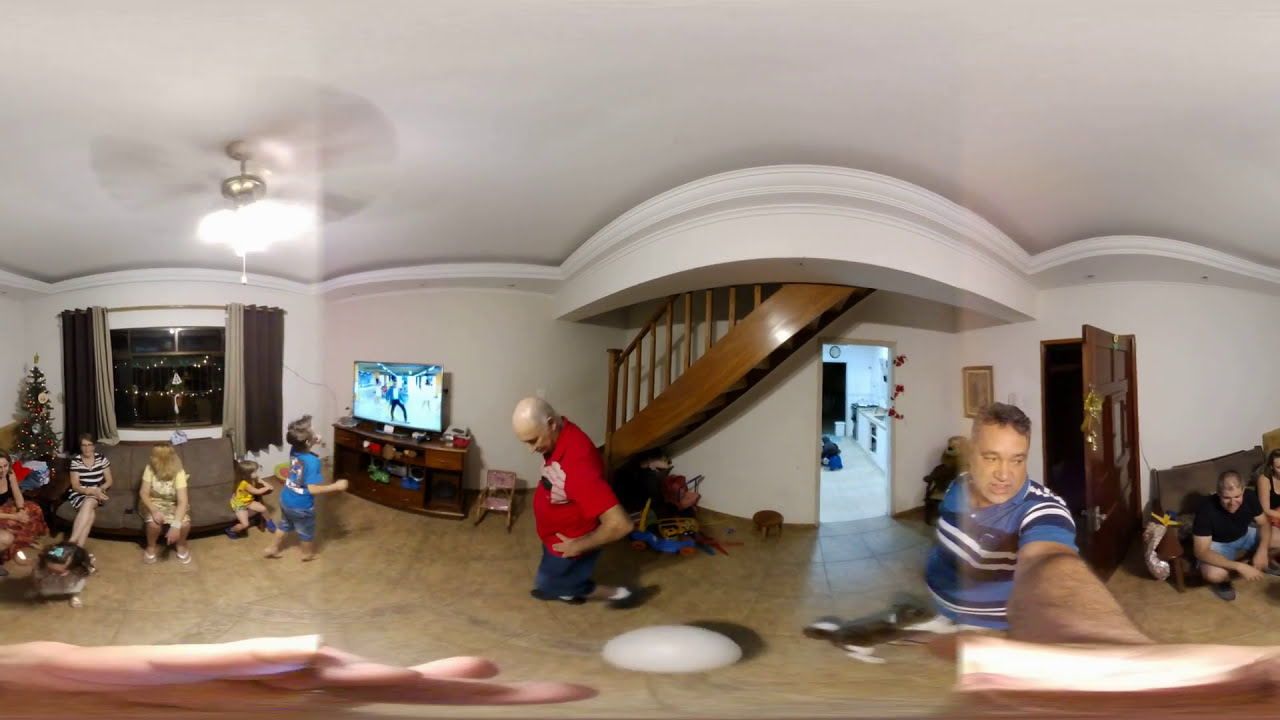The image is a 360-degree shot of a living room taken in the evening or at night, likely during Christmas time given the small green Christmas tree adorned with lights in the far left corner. The scene is a cozy family gathering where around six to eight people, including both adults and children, are present. The room appears distorted due to the lens, making the layout and spatial relations somewhat confusing, but the festive mood is palpable.

In the left part of the image, beneath a dark window illuminated by numerous small outdoor lights, sits a red sofa facing inward. Two women are seated on chairs with a small coffee table in front of them, while a woman wearing a red shirt, notably distorted with her legs appearing unnaturally short, sits centrally and looks to the left. Nearby, an elderly man in a white shirt is seen looking downward with his arms on his waist. 

Towards the center-left, two small boys dressed in yellow and blue are engrossed in a TV screen on a stand, which features another person. A man in a blue, black, and white striped shirt stands to the right, holding his arm out towards the photo's edge, with a small pet—either a cat or dog—next to him. 

The background showcases a wooden staircase with a curved banister leading upstairs along the wall, while an illuminated doorway reveals a kitchen. A white ball is centrally placed on the hardwood floor, enhancing the homely vibe. On the right side, an open wooden door is visible next to another brown sofa, where another man and woman sit. Overall, the image captures a warm, intimate family night with everyone casually enjoying each other's company and the television.